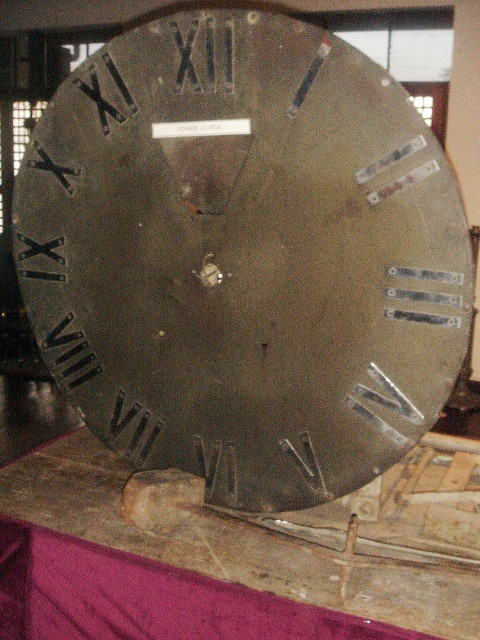The photograph features a large, weathered metal clock face adorned with Roman numerals. The clock is notably aged and tarnished, giving it a dingy and dark appearance. The center mechanism, where the clock hands would typically be attached, is visible but lacks the hands themselves. A partially legible white label with possible markings such as "tower clock" is affixed to the clock face. The clock is propped up on a wooden bench draped with a reddish-burgundy fabric. Bright light enters the scene through windows in the background, suggesting that the photo may have been taken indoors, possibly in a warehouse or exhibition space. Additionally, there seems to be a small rock placed in front of the clock, potentially for stability or display purposes. The entire setting gives the impression of an indoor display, emphasizing the clock's historical and decorative aspects.